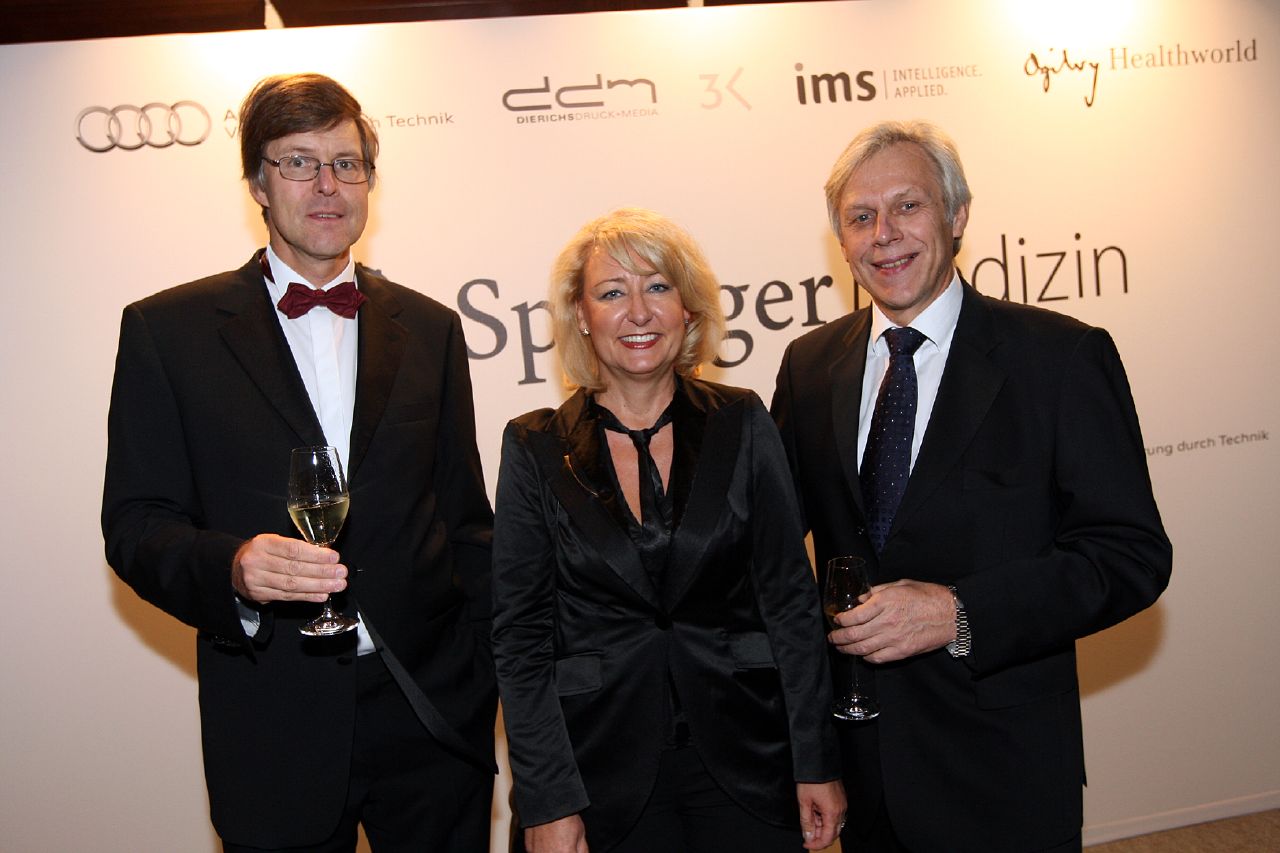The image is a photograph taken at an awards ceremony, featuring three Caucasian individuals standing in front of a white background adorned with various company logos such as Ogilvy, Health World, IMS, Intelligence Applied, Dearex Media, Technic, Audi, DDM, and 3K. 

From left to right:
- The first individual is a very tall man with sharp brown hair, glasses, and a red bow tie paired with a black suit. He holds a glass of wine in his right hand.
- In the middle stands a slightly shorter woman with blonde hair, dressed in a velvet black coat and a black tie, with her hands at her side. She appears to be in her 60s.
- On the right is another man with gray hair, also likely in his 60s or 70s, wearing a black suit and a blue tie. He holds a glass of wine in his left hand.

All three individuals are smiling and posing formally for the picture, suggesting it is taken at a significant and formal event, possibly an awards ceremony. The colors in the image are predominantly black and white, with noticeable accents including the red bow tie, blue tie, and the yellow tint from the wine in their glasses.